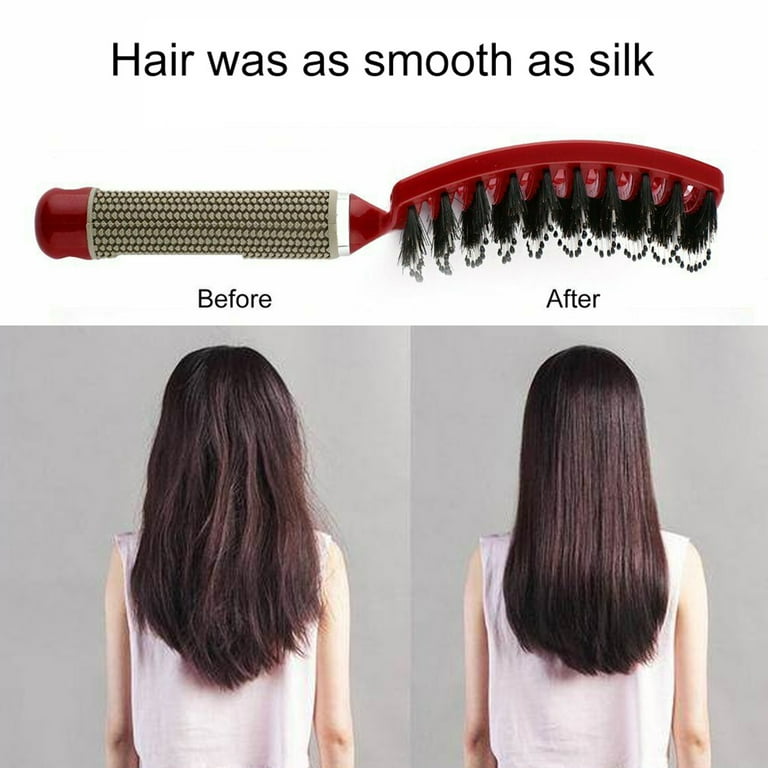This colored photograph is an advertisement for a maroon hairbrush with a tan handle and black bristles. The advertisement is divided into three sections. At the very top, bold black text proclaims, "Hair as smooth as silk." Below the text, the hairbrush itself is featured prominently, showcasing its distinctive curve and plastic construction. The bottom half of the advertisement features a before-and-after comparison of the same woman with long black hair and wearing a sleeveless white top, viewed from the back. The left side, marked "Before," shows her hair frizzy and unkempt, while the right side, labeled "After," displays her hair perfectly combed, smooth, and neat. This visual narrative emphasizes the transformative effect of the hairbrush, promoting the idea that it makes hair silky and presentable.